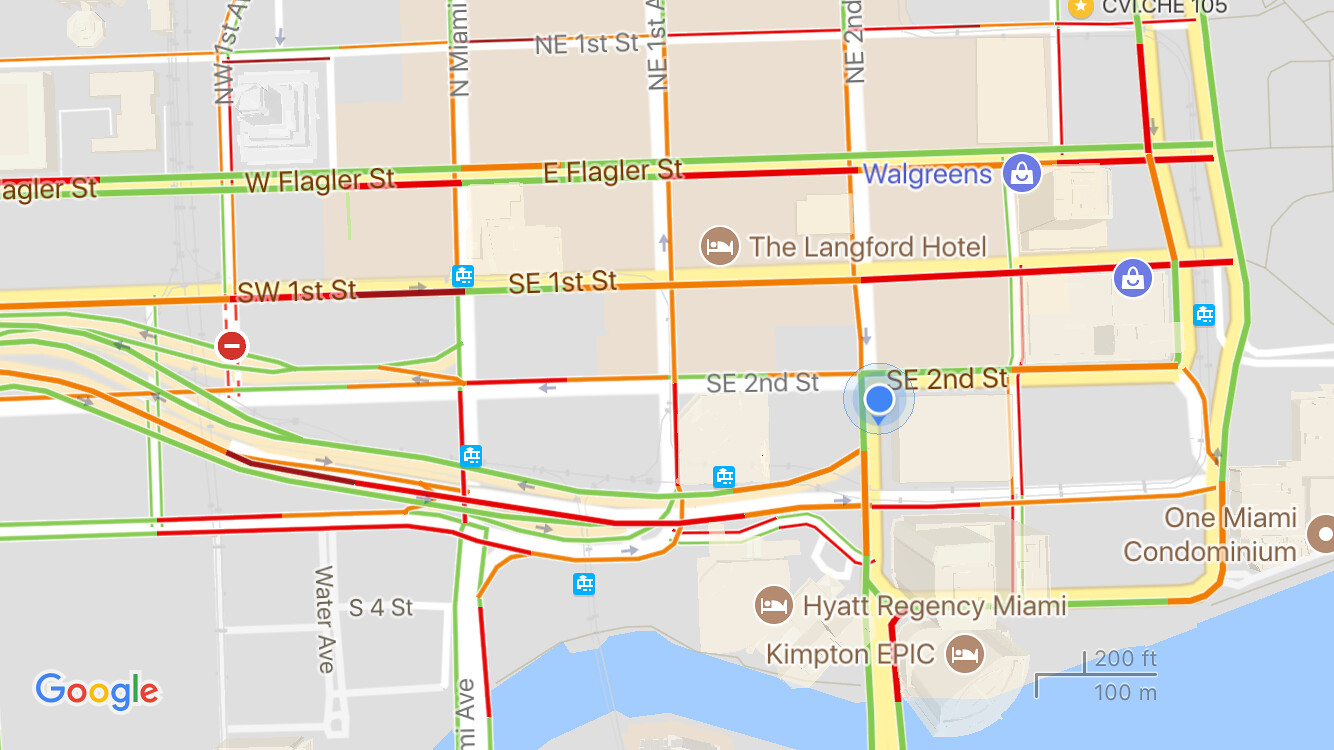This image depicts a high-quality screenshot of a Google map, evidenced by the "Google" logo in the bottom left-hand corner. The map, which is a standard colored illustration rather than a street or satellite view, predominantly features a beige and gray theme, intersected by various streets and highlighted lines in green, yellow, orange, and red. The map focuses on a section of downtown Miami, identifiable by landmarks such as the Hyatt Regency Miami, One Miami condominium, the Langford Hotel, Kimpton EPIC Hotel, and a nearby Walgreens. Southeast 2nd Street, marking the location with a blue circular dot, signifies where the screenshot was taken. Notable streets include East Flagler Street, Southwest 1st Street, and Southeast 1st Street, with a visible waterway in the right-hand corner. The map layout suggests a grid-like street arrangement, and despite the presence of highways, their specific designations are not clear in the image.